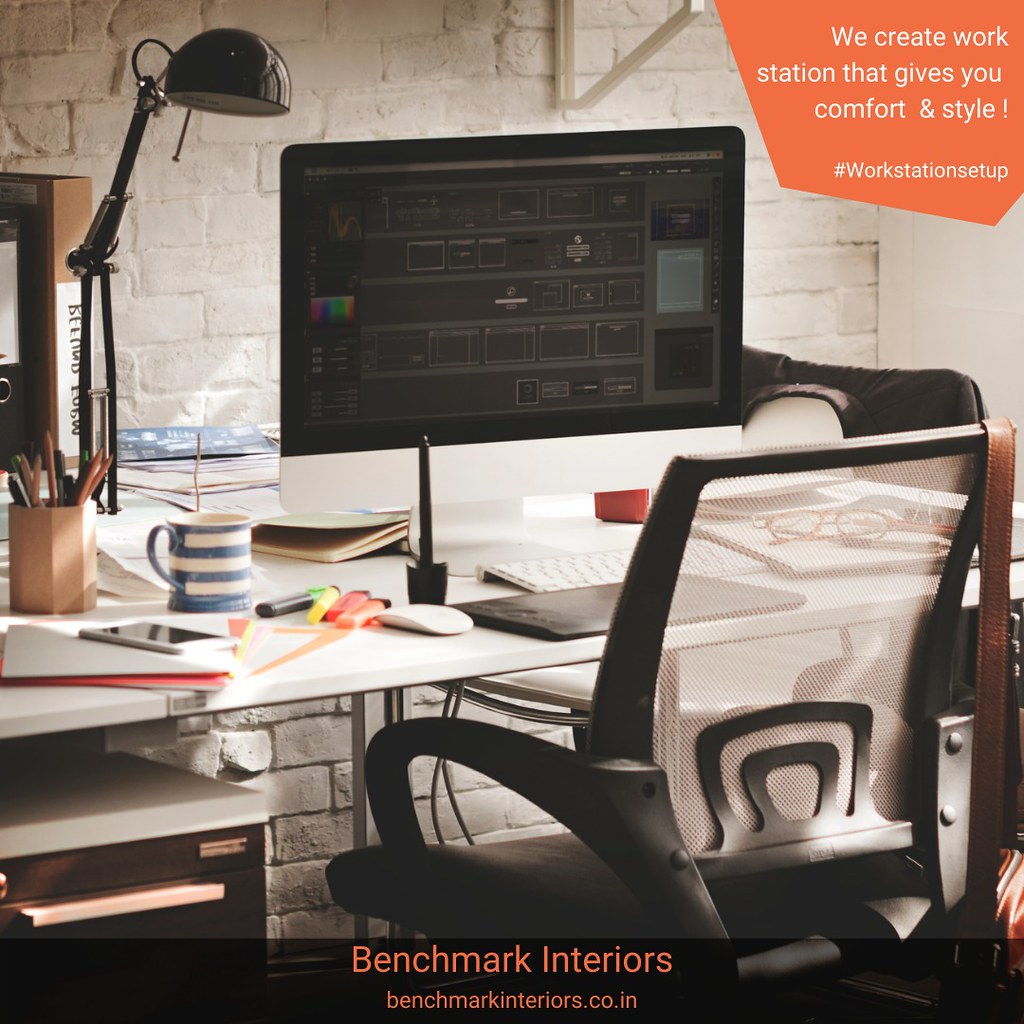The image depicts a meticulously organized, predominantly white office setup characterized by clean lines and minimalist design. Central to the scene is a sleek white desk cluttered with various essentials, including a blue and white mug, several highlighters, a keyboard, and a laptop. A striking feature is the modern black desk chair with a see-through backrest positioned in front of the desk. Adding to the functionality and style of the space is a black lamp subtly lifting over the desktop. An orange sign on the right corner of the image bears the slogan "We create workstation that gives you comfort and style" in white lettering, followed by the hashtag #workstationsetup. The bottom of the image prominently features the branding "Benchmark Interiors" along with the website "benchmarkinteriors.co.in". Altogether, this setup illustrates an inviting, well-organized office environment crafted for both comfort and productivity.